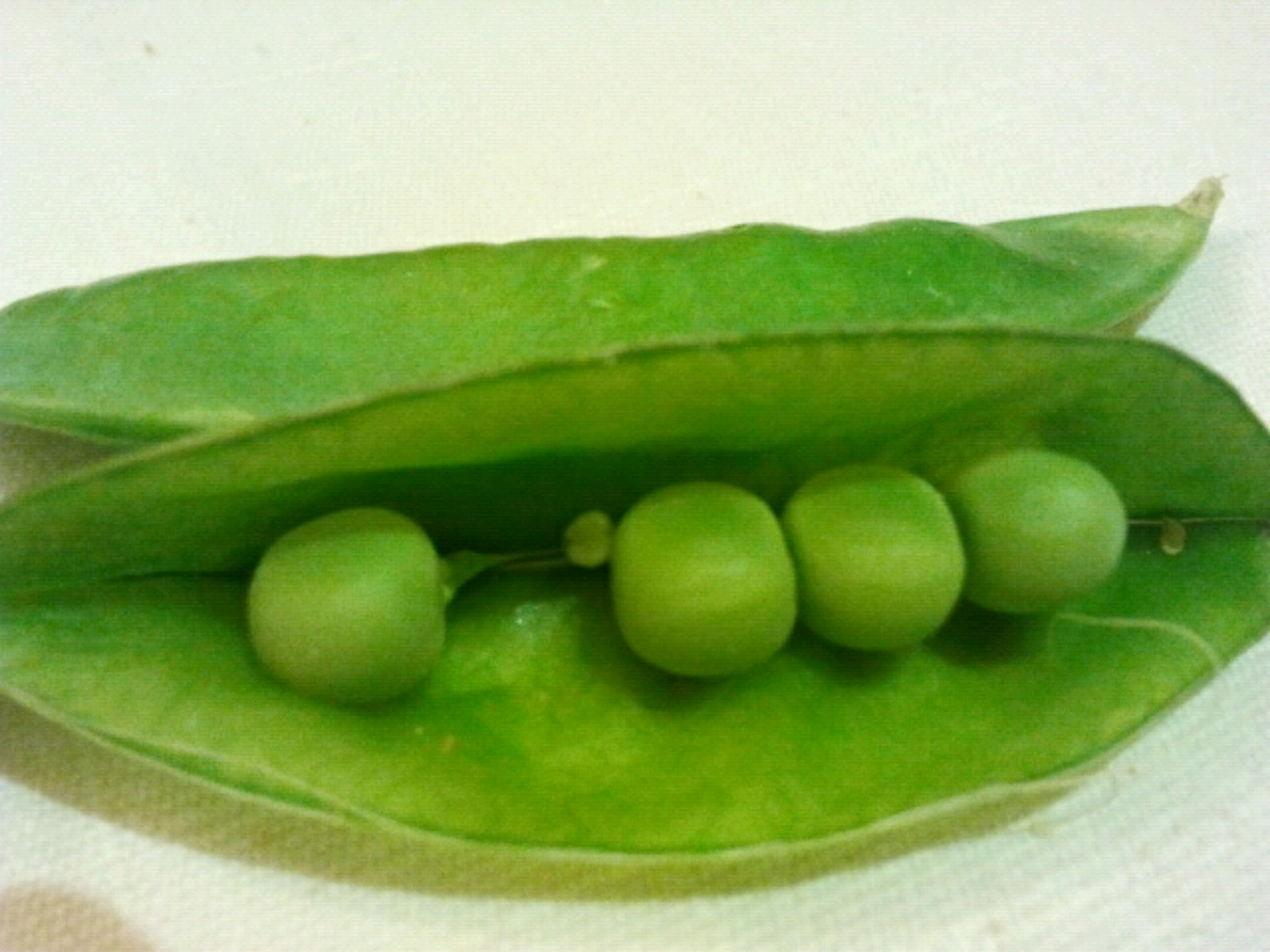The image is a detailed macro shot of two sugar snap pea pods on a textured white surface that resembles cheesecloth or a soft paper towel. The peas exhibit vibrant greenery with subtle whitish tips. The top pod is sealed and whole, showcasing its smooth, unbroken skin. Below it lies the second pod, which has been sliced open along its rounded edge, revealing four mature, bright Granny Smith apple-green peas inside. The peas are arranged in a row, with three clustered together on the right and one separated on the left. The white background, characterized by its soft, tightly woven fabric-like texture, also shows a faint thumbprint shadow on the bottom left, adding depth to the composition.